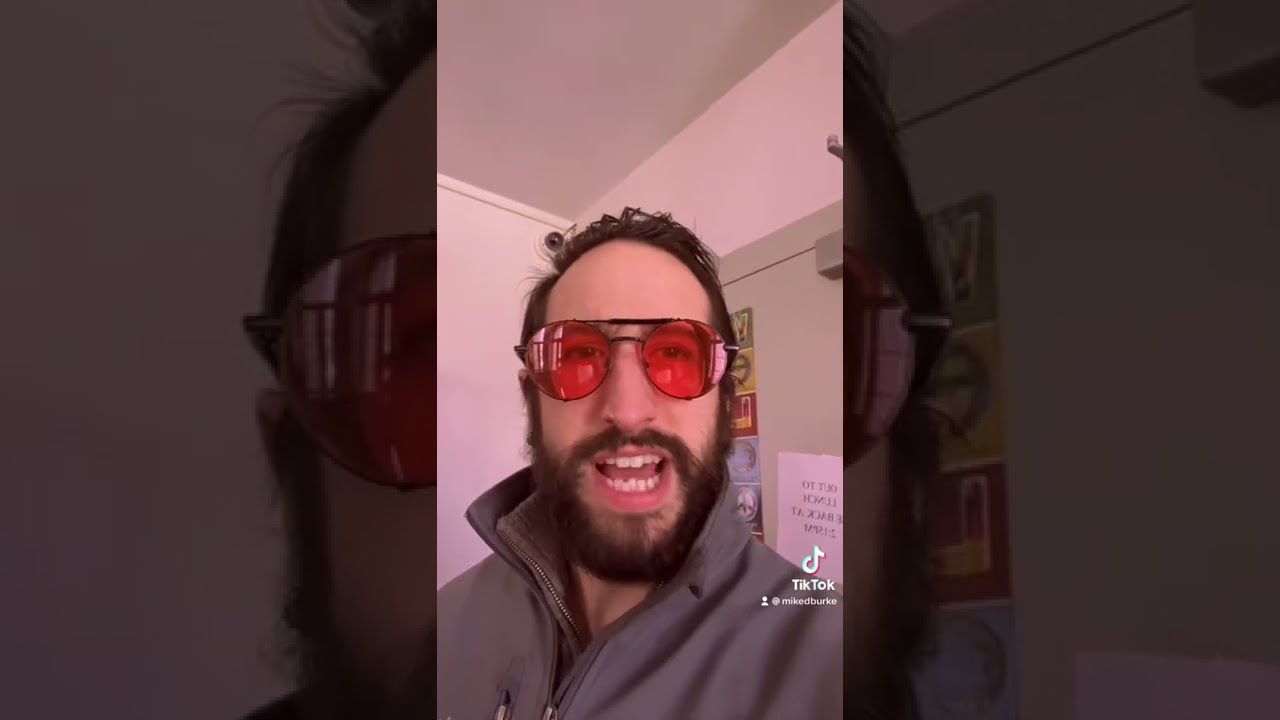The image is a three-part composite, with a well-lit central portion depicting the full head-and-shoulders portrait of a man. The outer portions are closely zoomed-in, lateral views of the same image. The man appears to be a TikToker, likely in his late 20s or early 30s. He has a receding hairline with short brown hair, a full brown beard, a mustache, and is wearing distinctive sunglasses with an orange or pink tint and a metal bar over the top of the nose piece. He is seen smiling with his teeth visible and his mouth slightly open as if speaking. He's clad in a gray zip-up jacket over another zip-up sweater. The background features a door with a greenish hue, adorned with a white sign with black text and a poster with pictures. At the top of the door, there’s a metal hydraulic hinge. Other details in the room include white walls and ceiling. The TikTok logo and more text in white font are visible on his shoulder. The overall tone of the image has somewhat reddish hues while the sides contain enlarged, grayed-out segments of the same facial portrait.